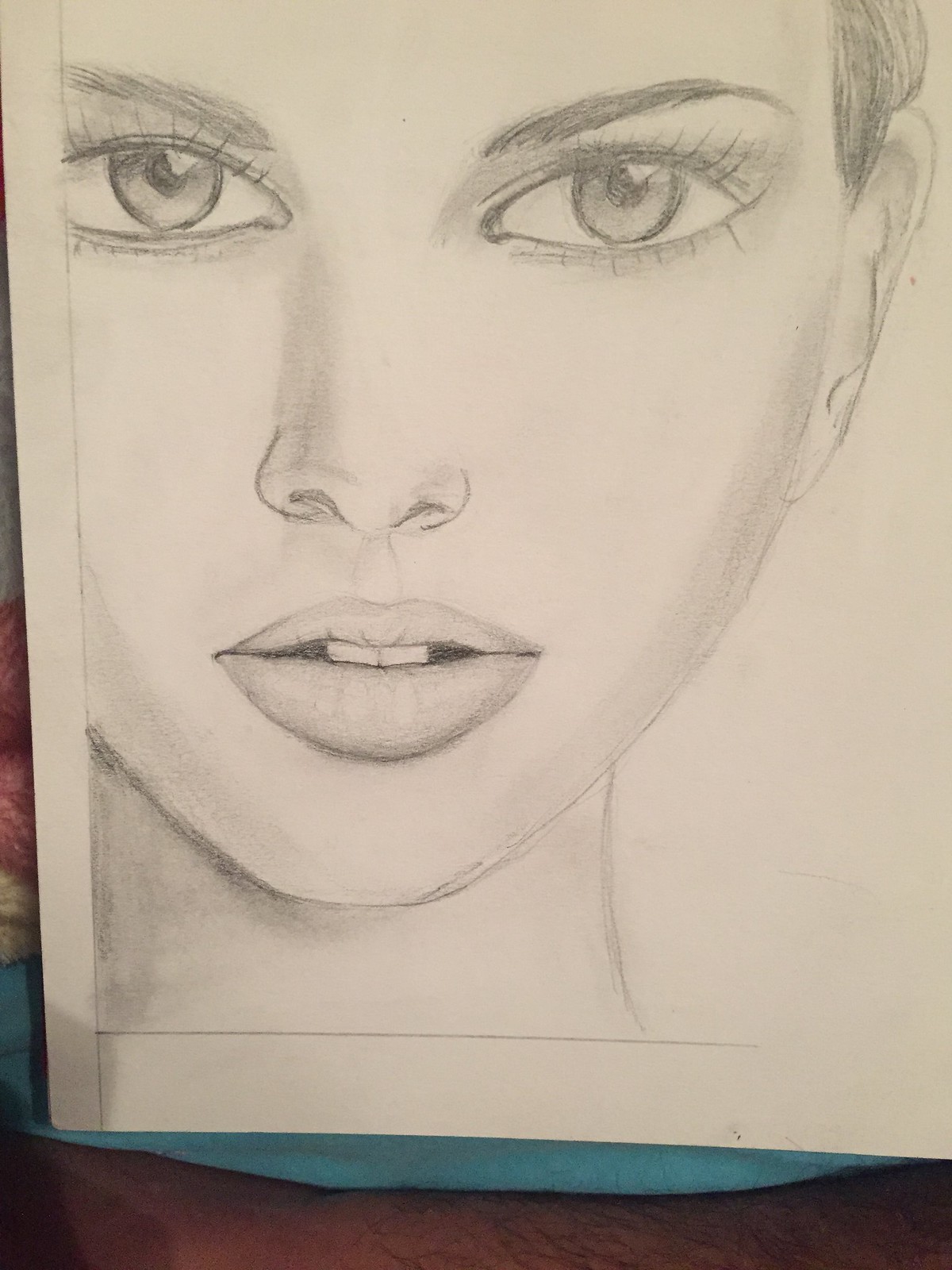This portrait-format penciled sketch, depicting a young Caucasian woman in her late teens to 20s, is executed on a sheet of upright white paper. Rendered in graphite pencil, its details showcase the artist’s experience and skill. The close-up view captures her face from the chin up to slightly above her eyebrows, and from her left ear to nearly the outer edge of her right eye. Her large, reflective eyes, slender nose, and plump lips lend her a relaxed, semi-serious expression. The limited hair visible is above her ear, while the shading accentuates her neck and ears, bringing additional depth to her proportionate features. Despite some cut-off features on the right side of her face and midway through her neck, the drawing’s refined lines and potential preparatory indications suggest a thought towards future framing.